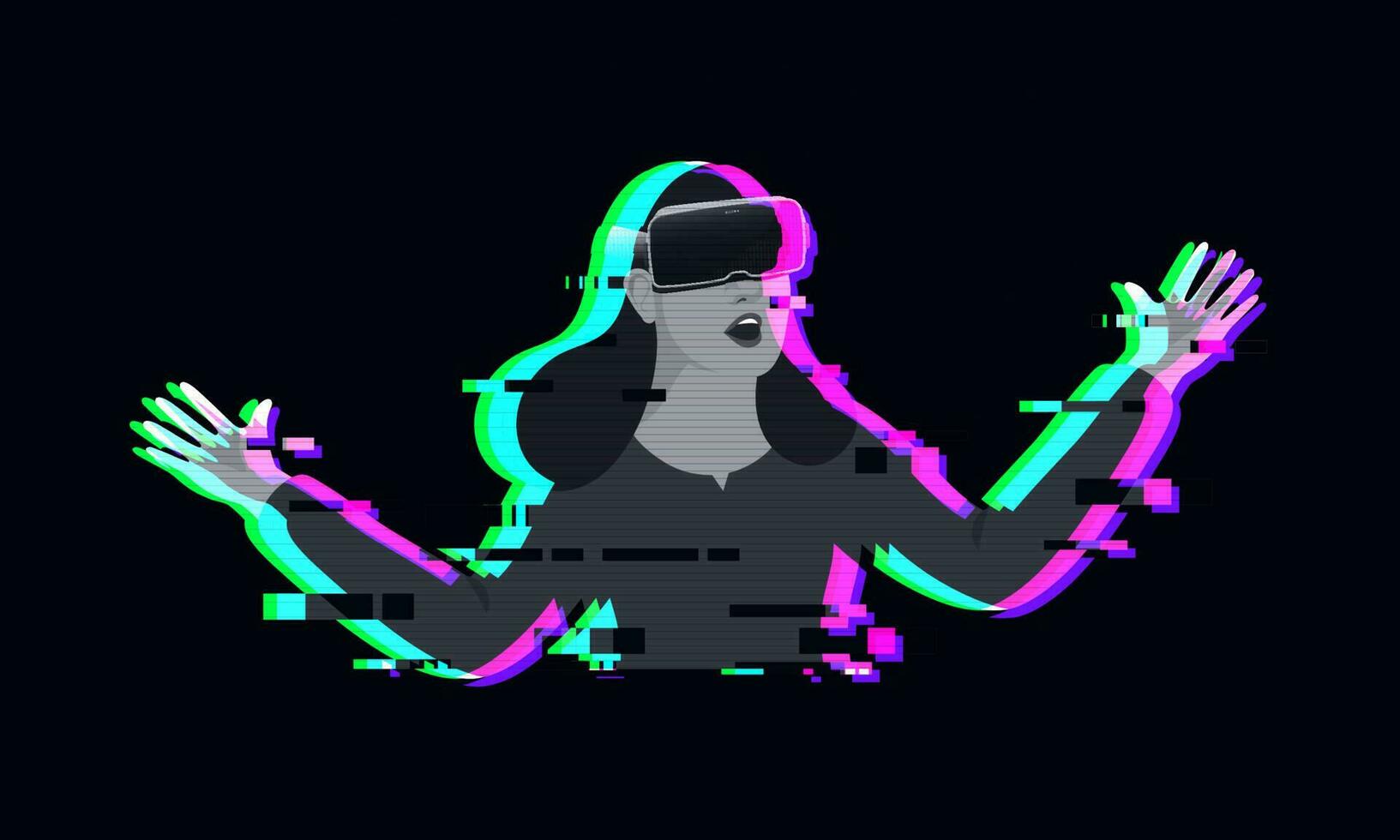This captivating digital illustration depicts a woman immersed in a virtual reality experience. Set against a stark black background, the woman, illustrated from the chest up, commands the center of the image. She is wearing a dark gray long-sleeved top with a small V-cut around the neck, and her long, black hair flows around her. Her most striking feature is the rectangular VR headset that covers her eyes, leaving her mouth open in a vivid expression of awe, revealing her top teeth. Her arms are outstretched to her sides, as if reacting to the immersive digital environment she perceives through the goggles.

The illustration possesses a distinct glitchy, cyberpunk aesthetic, accentuated by bright green, aqua, and pink outlines that trace the woman's form. These vibrant borders, particularly the teal green on her left and neon pink on her right, overlap to create an illusion of digital artifacts and missing pixels, reinforcing the futuristic, glitch-like effect. The combination of these elements, along with the woman's monochromatic skin tone, creates a sense of dynamic movement and a visually arresting representation of virtual reality in a modern digital age.